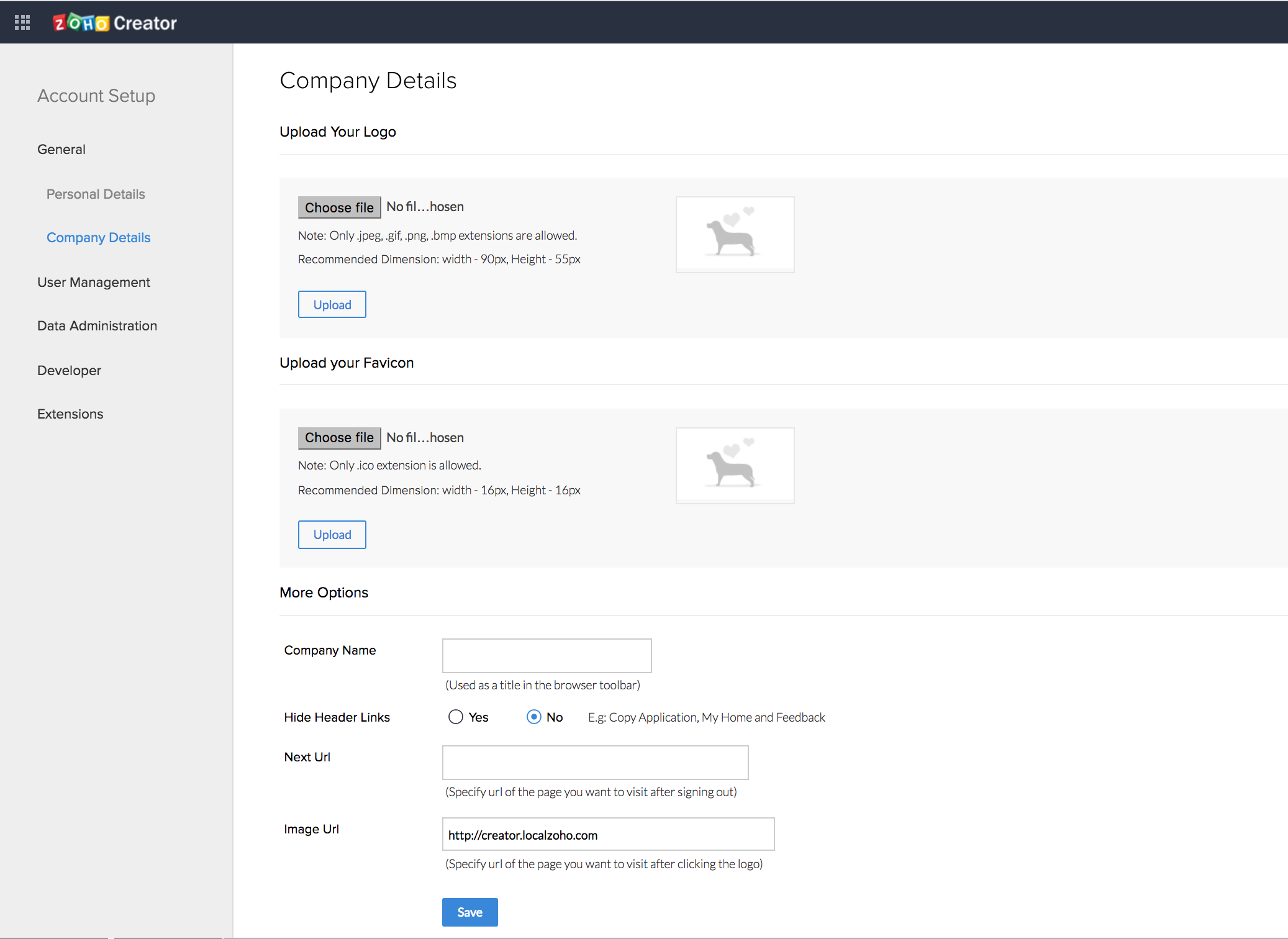In the upper left corner, the text "ZOHO Creator" is displayed, with the letters "Z," "O," "H," and "C" each housed in individual colored blocks—red, green, blue, and yellow, respectively, resembling children's building blocks. This is all set against a black strip running across the top of the interface. To the far left, a grid of nine small squares forms a larger square icon. There's a vertical gray stripe on the left side, serving as the navigation panel. It lists the following menu options: Account Setup, General, Personal Details, Company Details (highlighted in blue as the current page), User Management, Data Administration, Developer, and Extensions.

The main content area displays the "Company Details" section, offering options to upload a company logo with an input field labeled "Choose File," which shows "No file chosen" by default. Below this, there is a note specifying that only JPEG, GIF, and PNG bitmap extensions are allowed, with recommended dimensions of 40 pixels in width and 55 pixels in height. A blue-edged upload button with blue text on a white background sits beneath this information. Following is an option to upload a favicon, featuring another "Choose File" input field with "No file chosen" displayed. A note specifies that only ICO file types are accepted, with recommended dimensions of 16x16 pixels.